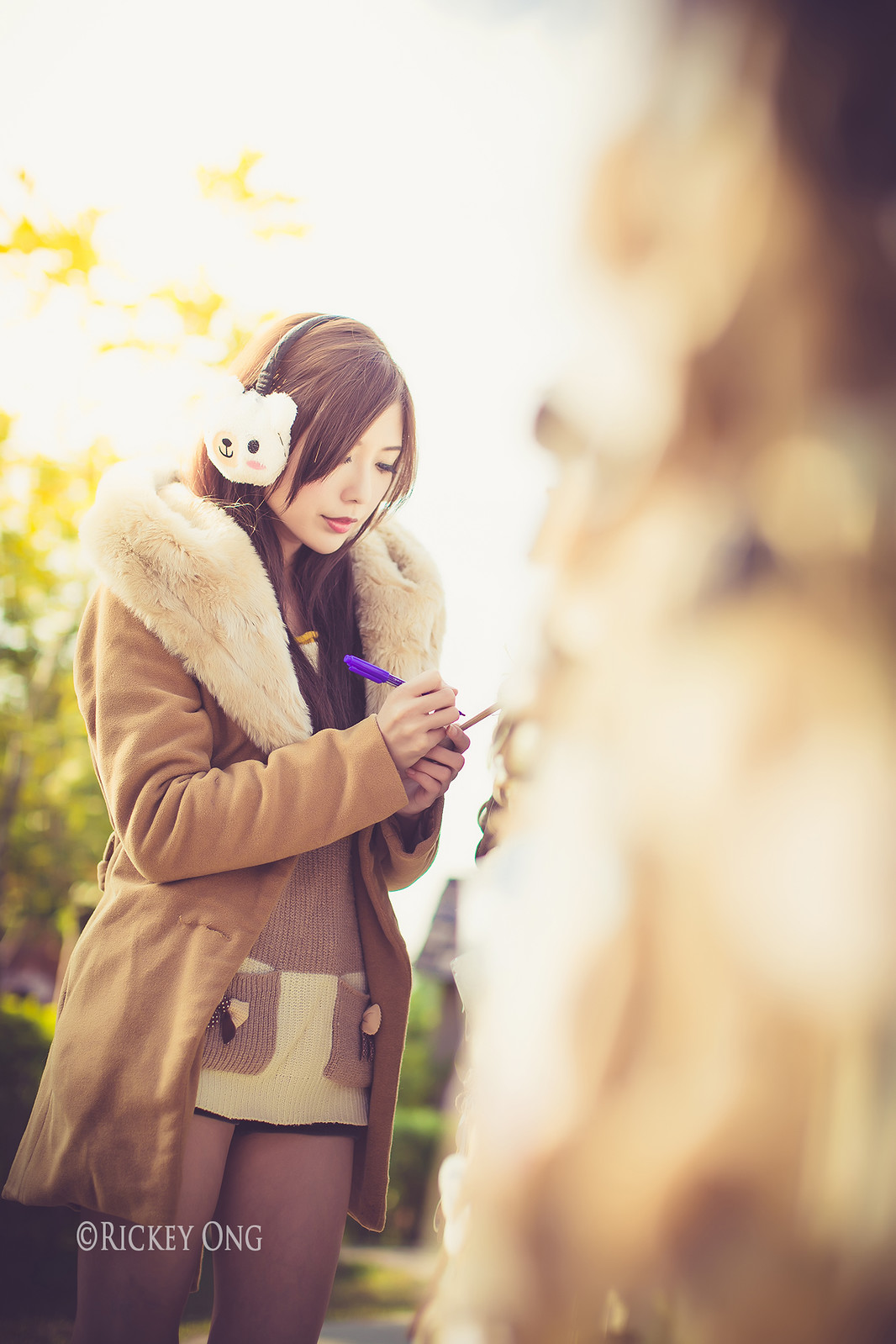The image captures a young woman standing outdoors, likely in a park, with trees or greenery softly blurred in the background. She is looking down, focused on writing something on a small notepad. She holds a purple pen in her hand. The woman is dressed warmly, wearing a brown winter coat with a large fur collar that extends to mid-thigh. Underneath her coat, she has a tan-brown sweater paired with matching pants. Earmuffs resembling the head of a white bear cover her ears, and she has long dark hair. On the right side of the image, a tree trunk is barely visible, blurred and out of focus. In the bottom left corner, there is a copyright symbol alongside the name "Rikki Ong."